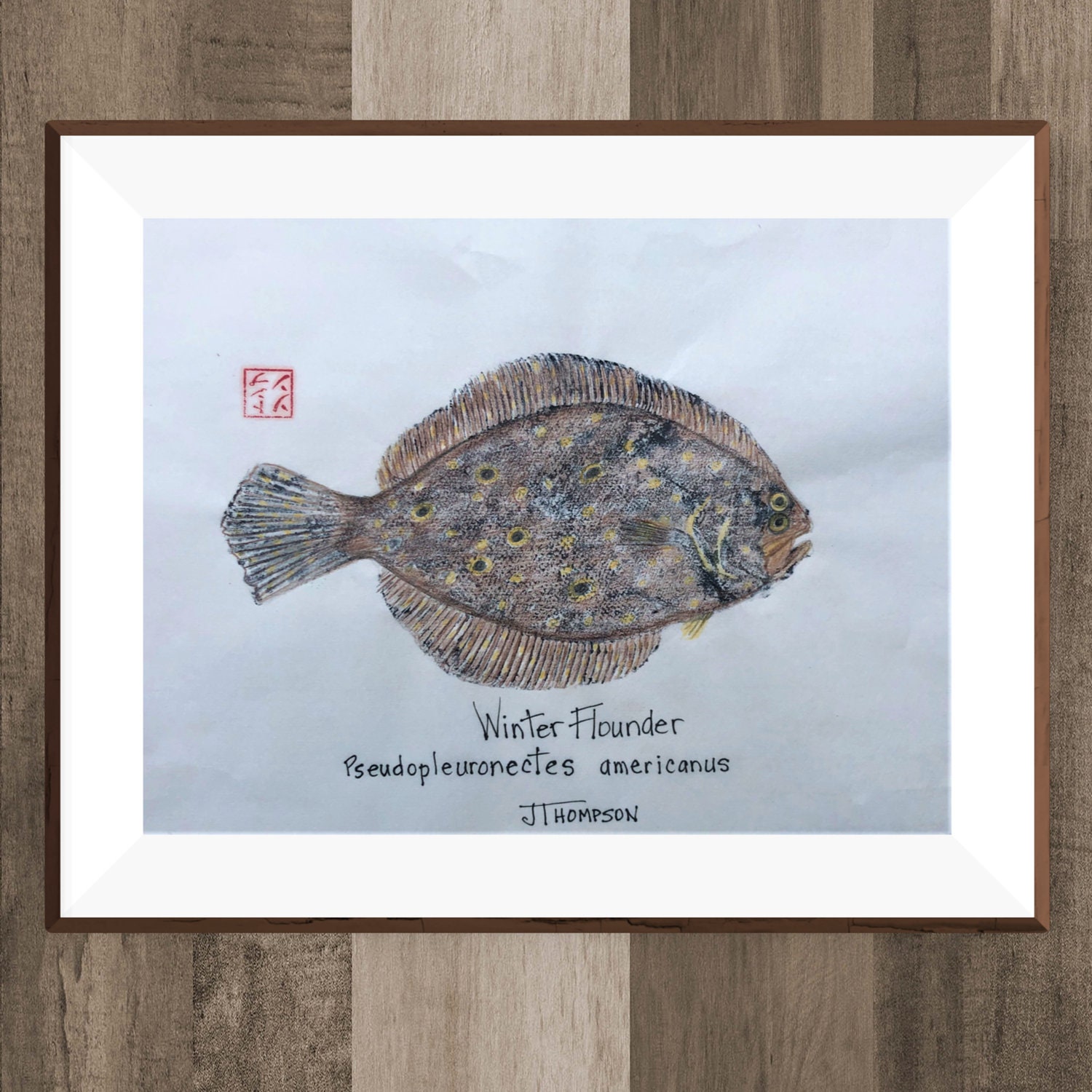The image depicts a framed drawing of a winter flounder, created by J. Thompson, prominently hung on a vertically-paneled wooden wall. The wall features slats of wood in varying shades of light brown, dark grayish brown, and a beach-like hue. The artwork itself is encased in a thin brown frame with a white mat. The fish, positioned centrally on a white background within the drawing, has a round body with a distinctive coloration: predominantly gray with yellow spots that have black centers. The fins, which extend from the top and bottom of the body, share the same color pattern. The tail is silver with yellow spots, and the face of the fish is brownish with a distinctive yellow eye featuring black dots. Text below the fish identifies it as a "Winter Flounder" with its scientific name, "Prosupera kineticus americanus," and the artist's name, "J.T. Thompson." Additionally, a small red emblem is stamped onto the picture. The fish is depicted with a spiny dorsal and lower fins, a large tail, black spots, and an open mouth, facing toward the right against a blue background.